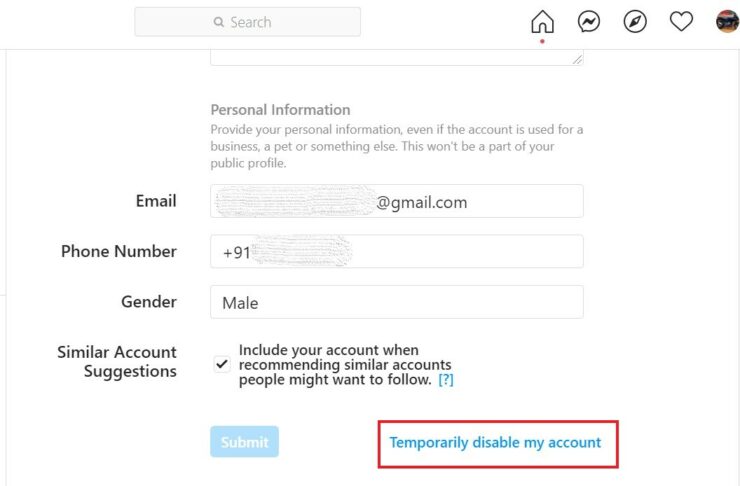The image depicts a user interface for entering personal information on a platform. At the top left, there is a light gray search bar. On the top right, there are several icons: a house, a bar with a zigzag or a bubble with a zigzag through it, a heart, a profile photo, and an element that looks like it could be a compass.

The main form is dedicated to inputting personal information, which can be used even if the account is intended for business or other purposes, such as for a pet. A note clarifies that this information will not be part of the user's public profile.

The form includes sections for email and phone number, with parts of the entered information blurred out for privacy—specifically, the part before "@gmail.com" in the email address and the digits following the country code "+91" in the phone number.

There is also a gender selection marked as "Male" and an option for similar account suggestions, which is selected. This option reads, "Include your account when recommending similar accounts people might want to follow."

At the bottom, there is a blue "Submit" button. Additionally, there is text that reads "Temporarily disable my account," surrounded by a red rectangle, likely highlighted for instructional purposes to draw attention to this option.